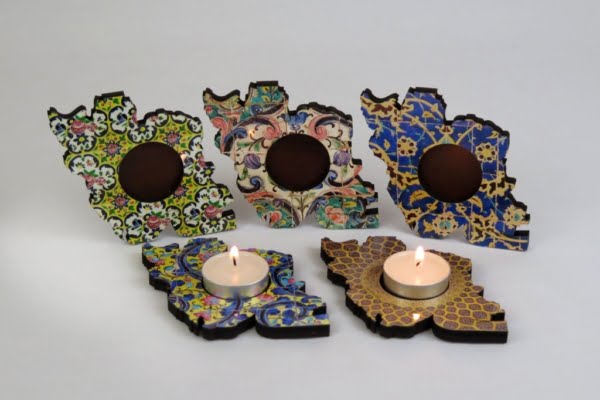The image features five uniquely shaped yet uniform ceramic votive candle holders, displayed against a gray background. Each holder has a distinct pattern and color scheme, primarily using greens, blues, beiges, pinks, and golds. The bases are painted with abstract designs, with some featuring white flowers against green backgrounds, while others showcase shades of tan, purple, and red. The central insets of the holders are round and dark, indicating where votive or tea light candles are placed, and are slightly recessed. Two of the holders contain lit candles, their flames visible, adding a warm glow to the scene. These holders, which are small and visually striking, are reminiscent of coasters but designed specifically for displaying candles. Notably, the product presentation does not include any contact information or company branding.